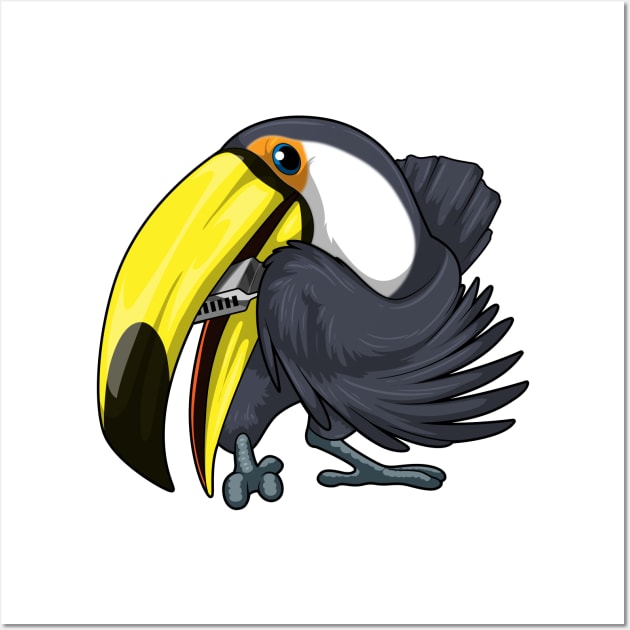This detailed digital drawing depicts a cheerful toucan with predominantly black feathers, playing a silver harmonica. The toucan, which may serve as a graphic design for a music logo, stands out with its long yellow beak that has a black tip and an orange edge. Its face features white feathers with an orange ring around its blue eye, suggesting a lively expression as it looks at the camera. The bird’s claws are gray, and it appears to be dancing, adding a playful element to the scene. The interior of its mouth, open as it blows the harmonica, has a dark pink hue. The background of the image is white, ensuring the vibrant colors of the toucan remain the focal point.